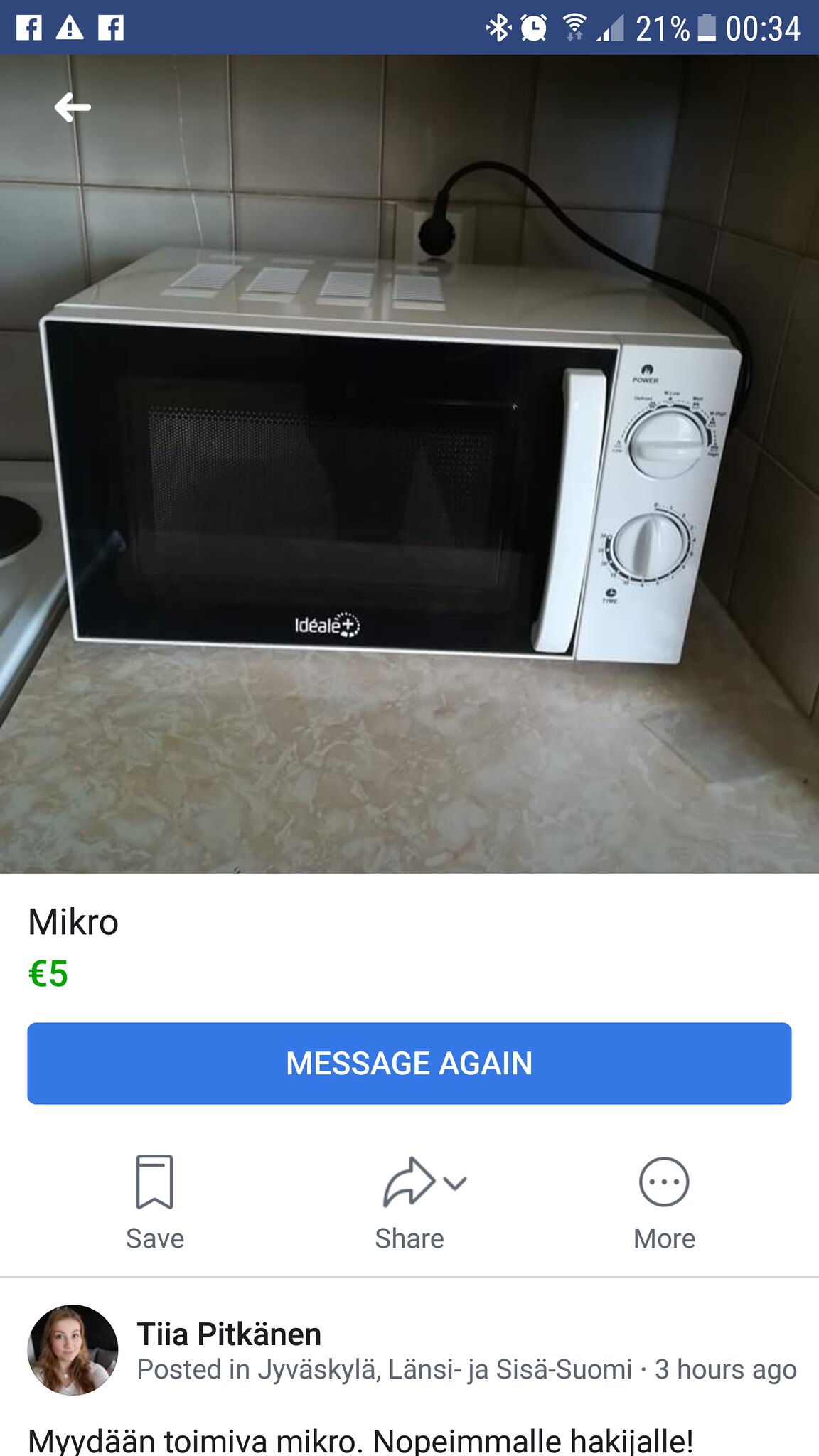This is a Facebook Marketplace listing for an older white microwave oven with a black door. The microwave, branded as IDEALE, features two knobs labeled "power" and "time." The listing includes a photo of the microwave and is captioned with "M-I-K-R-O 5 euros." Below the listing, buttons for "message again," "save," "share," and "more" are visible, represented by standard internet icons. The ad was posted three hours ago by a woman named Tia Picatson, with her profile picture showing a woman with brown hair. The Facebook interface is notably recognizable at the top, and the user's phone battery is at 21%. The ad appears to be written in a foreign language, possibly Swedish or similar.